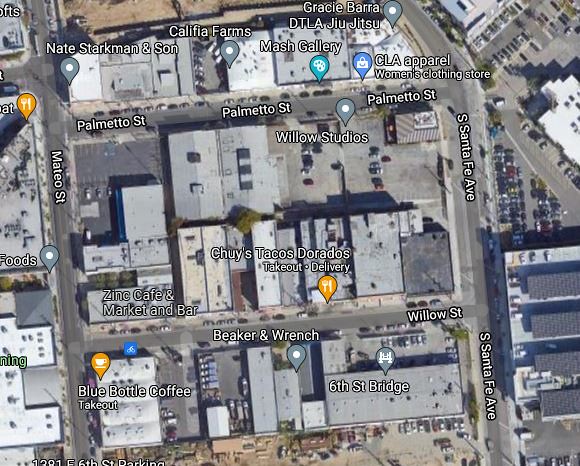This satellite photograph, potentially captured via a mapping software similar to Google Maps, offers a detailed aerial view of a densely built urban neighborhood. Centered around the intersection of Palmetto Street, Mateo Street, and South Santa Fe Avenue, the image highlights several notable landmarks and locations.

Prominent buildings and establishments are distinctly marked. Restaurants such as Chewy's Tacos and Blue Bottle Coffee are indicated by orange triangle icons, contrasting with the varied icons used for other types of businesses. Noteworthy landmarks include Nate Starkman and Son, Califia Farms, MASH Gallery, and Willow Studios, each marked with unique symbols.

The densely packed buildings display a variety of roof designs and colors, predominantly gray. Sixth Street Bridge is also visible, adding to the rich, detailed mapping of the area. The blue icon representing an apparel shop with a white shopping bag further adds to the intricate labeling of different venues within this urban landscape.